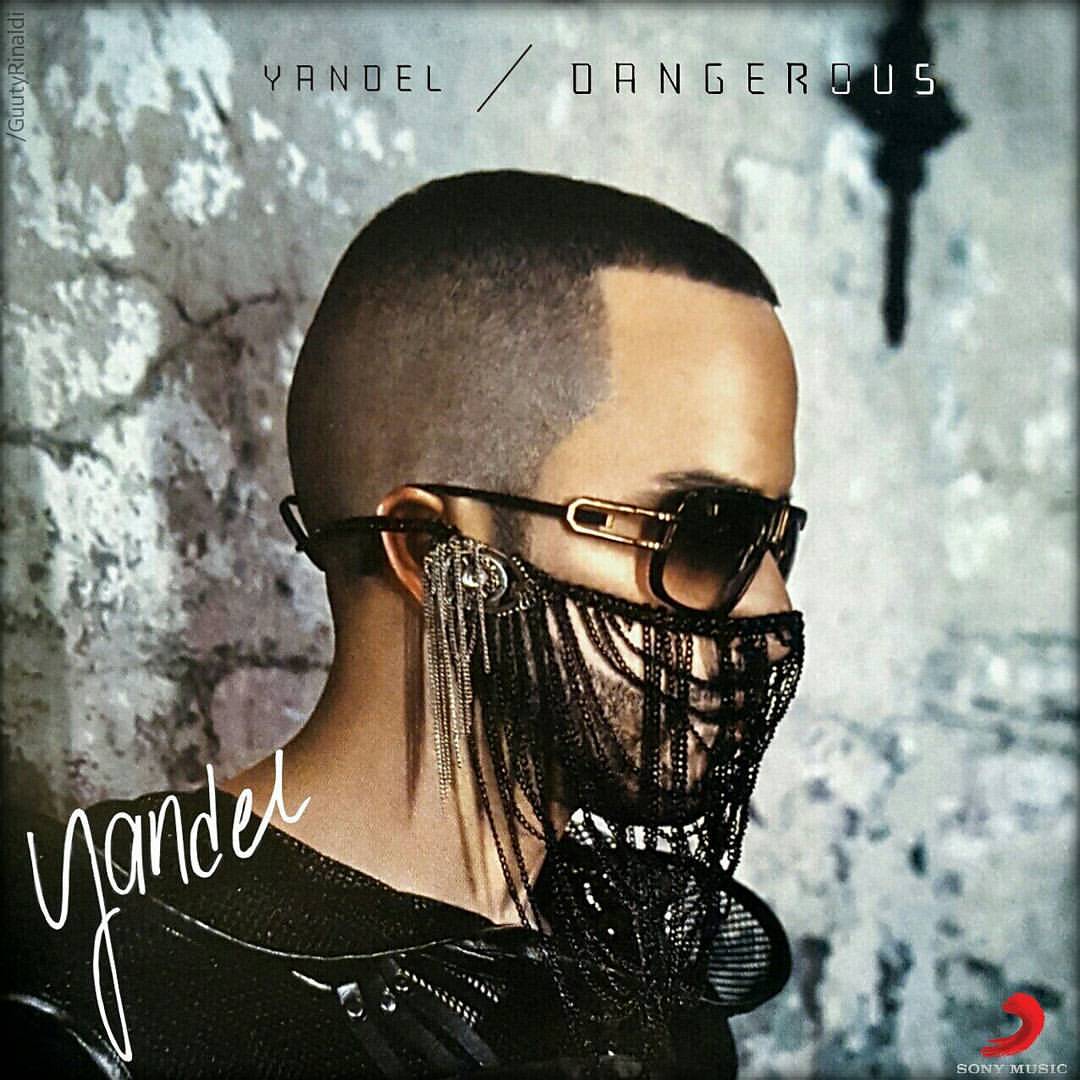This color photograph, possibly an album cover or promotional poster, features a young man in his right side profile, head and shoulders visible, standing against a backdrop that resembles a white and black marble stone wall. Dominating the top of the image are the words "YANDEL / Dangerous" in large print. The man, identified as Yandel by his signature in the lower left corner, is dressed entirely in black, including a black leather shirt or jacket. He sports very short dark hair and dark sunglasses, with a unique chainmail mask covering his nose and mouth, through which you can see his beard. This mask drapes down below his chin. Notably, a red symbol with some small, unreadable white writing adorns the bottom right corner of the image.